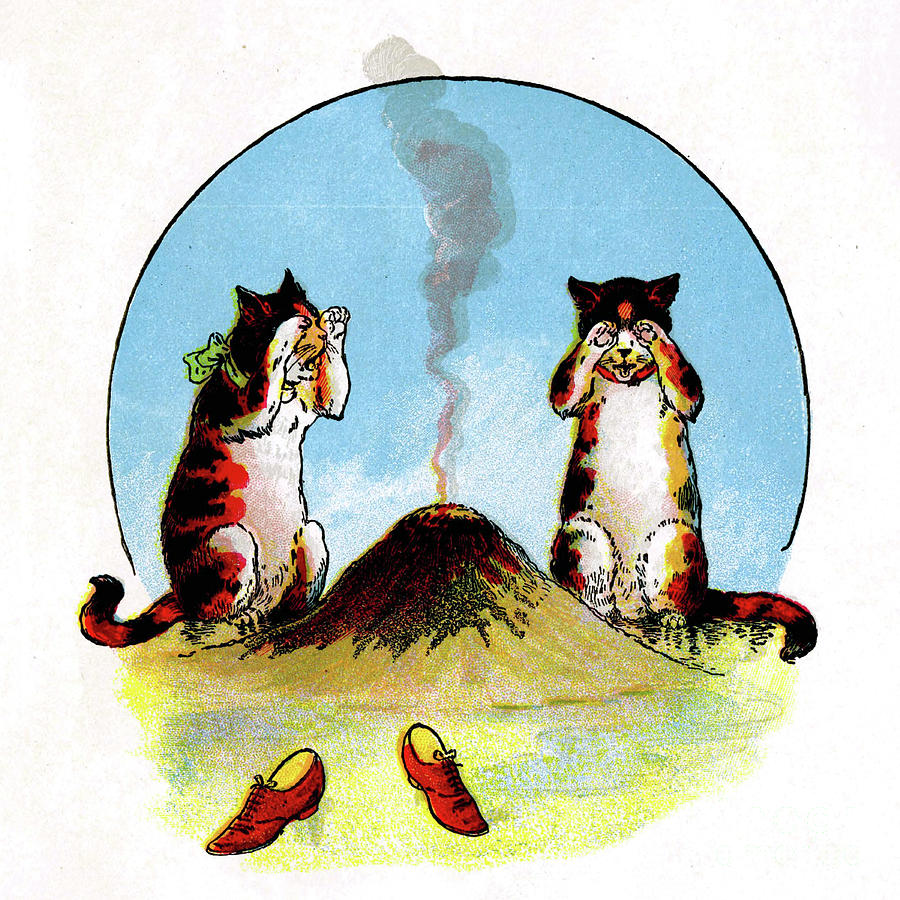This illustration features two cats sitting on their hind legs, covering their eyes with their front paws. Both cats have predominantly black and red fur, with white bellies and white undersides on their arms. One cat has a green bandana around its neck. They are positioned on either side of a small mound of dirt that emits a thin plume of smoke, transitioning from tan to dark brown and finally to gray. In the foreground, there are a pair of brown shoes with yellow insoles. The entire scene is set against a light blue sky, contained within a large black-outlined circle, possibly indicating a beach-like environment with lots of sand. The detailed elements of the scene highlight the cats' vivid emotions, the subtle background components, and the contrasting colors.